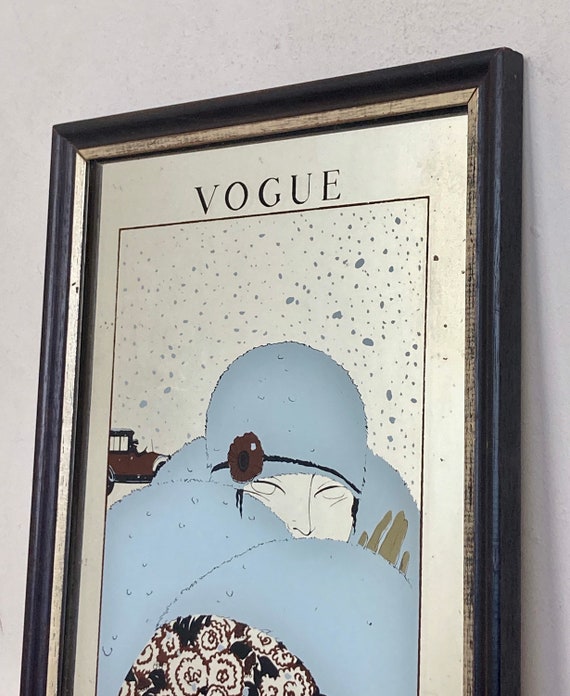The image depicts an Art Deco-inspired illustration on the cover of a magazine, which is elegantly framed inside a black wooden frame with a thin, weathered gold border. The magazine cover features the iconic "Vogue" title in black text at the top. Below that, a rectangle with a black border encloses the main illustration. The artwork shows the side profile of a woman, seemingly hugging someone, with her face partially obscured. She wears a baby blue, fuzzy hat adorned with a small brown flower decoration and a matching scarf. Her eyes appear to be shut as if she's in an intimate embrace. The backdrop of the illustration hints at a snowy scene, with flecks of white snow falling gently. In the background, there's a vintage car reminiscent of the 1930s or 1940s. The whole magazine cover leans against a pristine white wall, making the detailed framing and the delicate features of the illustration stand out prominently.